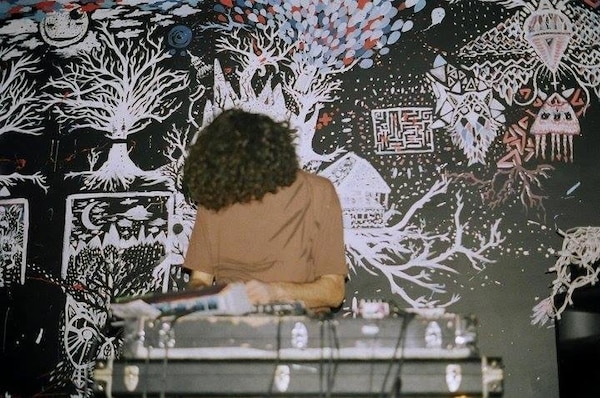In this detailed image, a person is positioned in front of a wall adorned with intricate artwork. The individual, seemingly a white male with long, shaggy, curly hair that obscures their face, is wearing a brown shirt and is focused downward, possibly setting up DJ equipment on top of two black cases that resemble guitar cases. The wall behind them is a canvas of various artistic elements: primarily white imagery interspersed with blues, reds, and pinks. Prominently, there are three detailed white trees whose branches and roots extend across the wall, as well as a maze and numerous other patterns. Additionally, the artwork includes a moon, mountainscapes, a fog-like effect, alien-like figures, and what seems to be an animal face or mask on the right side. Among the more vivid details, there are red and blue balloons seemingly being released from the trees, creating a lively and eclectic background scene for this music setup.